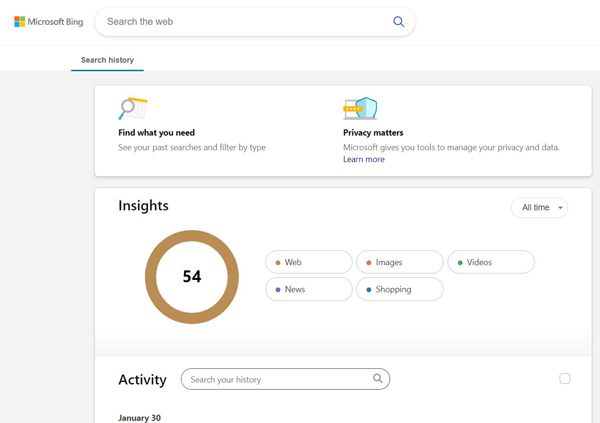In this image, we see a section of a webpage. In the upper left corner is the iconic Microsoft logo. Prominently displayed is a search bar labeled with the text "Search the web," accompanied by a magnifying glass icon in blue to its right. Below the search bar is a section titled "Search history," which is underlined in blue for emphasis.

Directly underneath, there is an icon of a magnifying glass followed by the phrase, "Find what you need. See your past searches and filter by type." This text is informative, suggesting users can review their previous searches and apply various filters. Below this explanation, there's a privacy-related note: "Privacy matters. Microsoft gives you tools to manage your privacy and data." The phrase "Learn more" is highlighted in blue, indicating it is a clickable link for more information.

At the bottom of this section are categories for different types of searches, each accompanied by a distinct color-coded circle. These categories are labeled as follows: "Web" with a brown circle, "Images" with an orange circle, "Videos" with a green circle, "News" with a purple circle, and "Shopping" with a blue circle. Additionally, the word "Insights" is followed by the number 54, hinting at the number of search insights available.